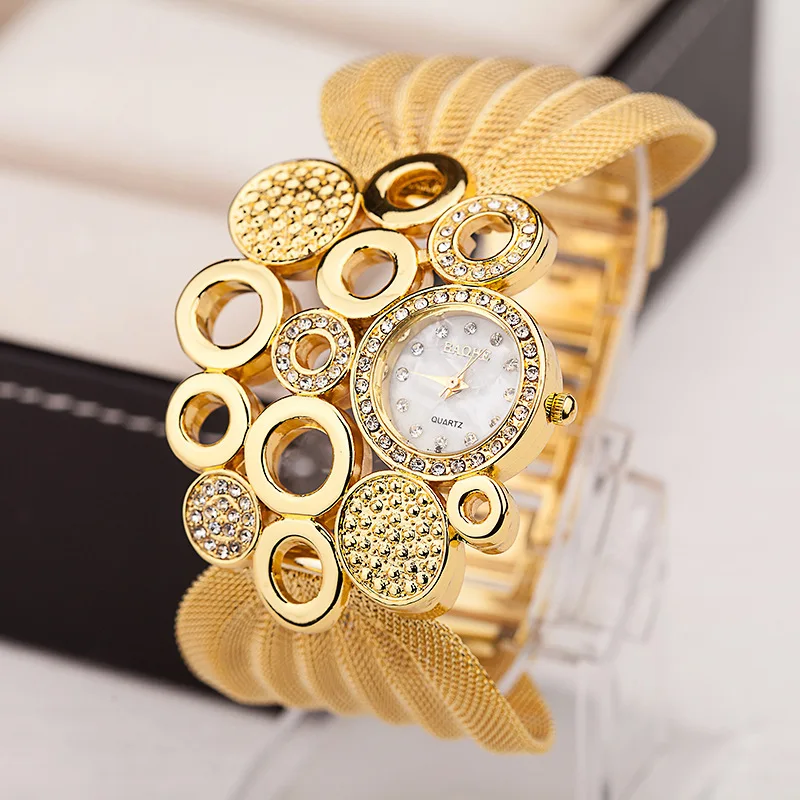In this close-up, overhead image, we see a very high-end, luxurious wristwatch displayed on a clear plastic holder. The background, which is out of focus, reveals a white surface and a blurry black box that suggests a leather-bound case with white stitching and white cushion rolls inside. The watch itself features an elaborate gold mesh band with thick gold webbing and intricate connections.

The watch face lies at the heart of a distinctive arrangement of twelve gold circles—three rows of four circles each—adorned with diamonds and some with hollow centers. Specifically, the left row consists of a solid gold circle with diamonds, followed by two hollow circles of varying sizes, and another smaller solid gold circle. The middle row features two hollow gold circles, one diamond-filled circular piece in the center, and another two hollow gold circles below. On the right side, a gold circle with diamonds and a hollow center is positioned above the watch face. The watch face itself is encircled by diamonds and features a gold bezel and knob. It has a white dial with diamond markers in place of numbers and the words "Bach, Bach, Quartz" inscribed on it. The overall aesthetic of the watch is very ostentatious, with extensive use of gold and diamonds, giving it an extremely fancy and expensive appearance.